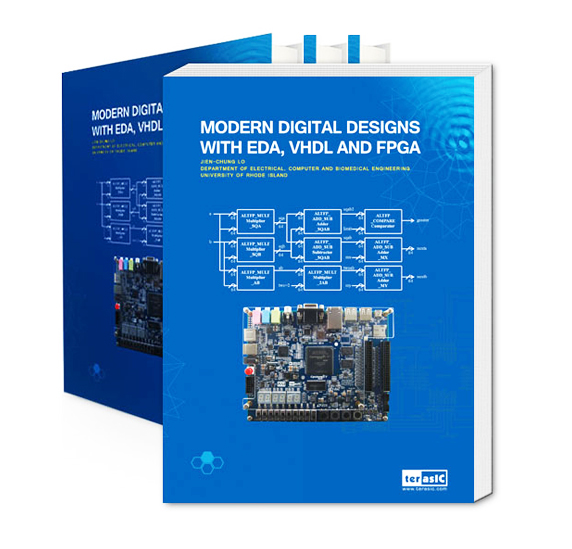The image depicts a set of four identical blue-covered books titled "Modern Digital Designs with EDA, VHDL, and FPGA." The front book is facing forward, showing intricate cover designs that include white illustrations of interconnected electrical circuitry and a gray computer motherboard populated with various colored electronic chips—yellow, blue, pink, red, black, and brown. Above the title, there's a detailed symbol featuring four hexagons, with the bottom three in blue shades and the top one in a lighter blue. Below the illustrations, the author is listed as Jincheng Lo from the Department of Electrical, Computer, and Biomedical Engineering, University of Rhode Island. On the bottom right, there is a barely readable web address starting with "TERASIC." The books behind are stacked at an angle, showcasing the blue borders of their covers.